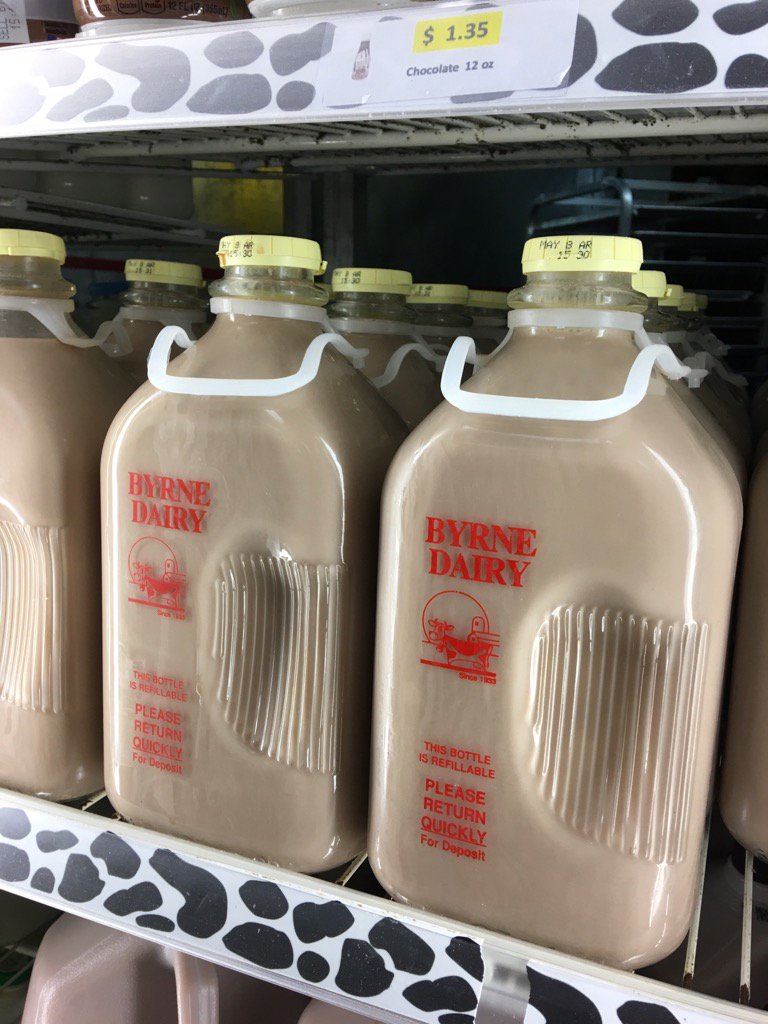The photograph captures the interior of a refrigerated dairy section in a supermarket, focusing on three rows of chocolate milk bottles. The top row is partially obscured by a price bar, indicating items such as "chocolate 12 ounce, $1.35." Beneath this, the middle and bottom rows display prominently large, refillable chocolate milk jugs, nearly gallon-sized. These jugs feature yellow caps and a distinctive white plastic handle for easy carrying. The bottles, made of glass, are etched with the label "Burn Dairy" in red letters, accompanied by additional red text that includes instructions like "please return quickly for deposit." The shelf itself has a white surface adorned with black, cow-like prints, reminiscent of a Holstein cow's spots, adding to the dairy-themed presentation.